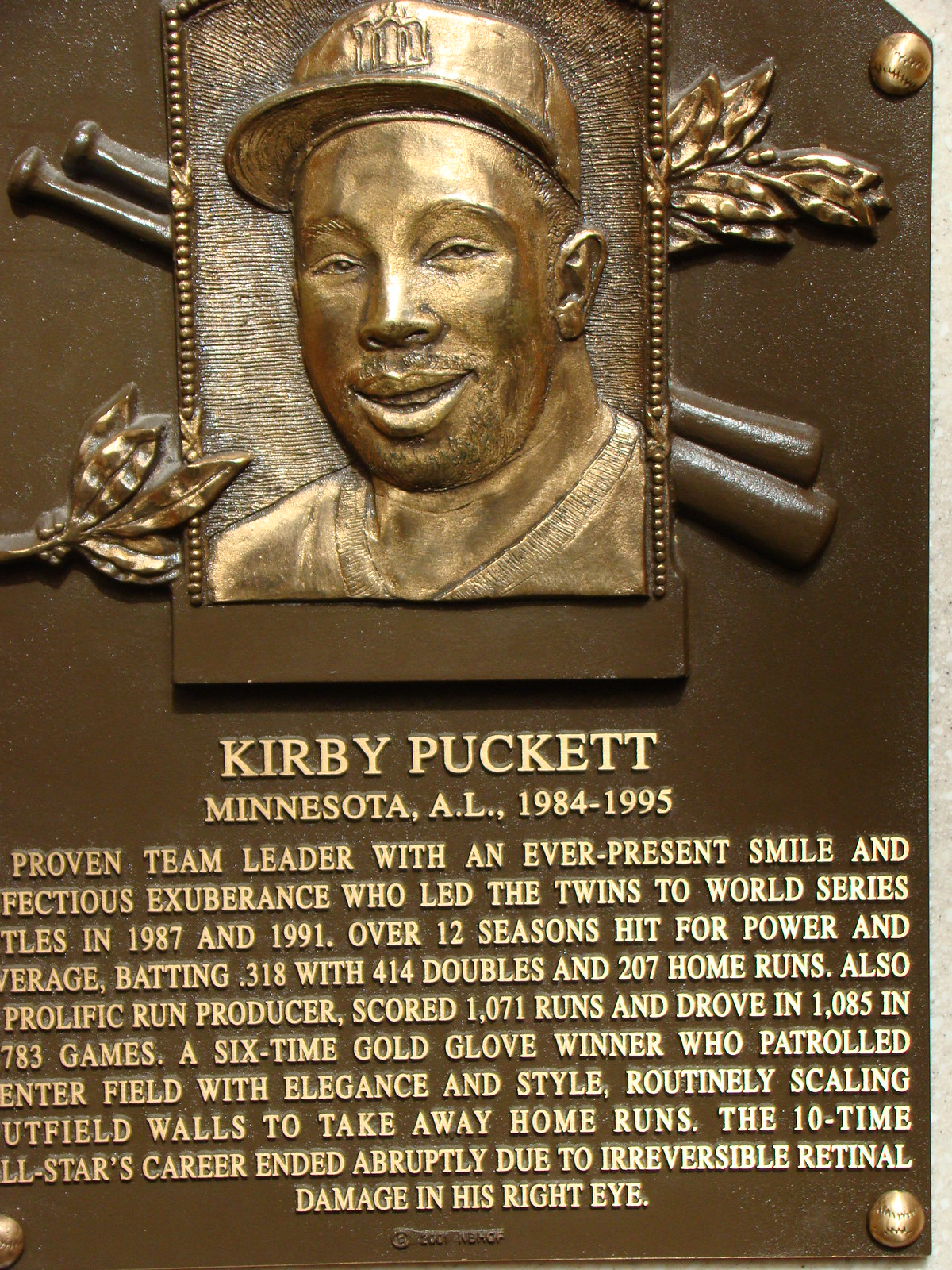The image is a color photograph of a bronze Hall of Fame plaque memorializing Kirby Puckett, a celebrated baseball player for the Minnesota Twins from 1984 to 1995. The plaque has a rich brownish metal finish, adorned with intricate details including tiny golden baseball-like screws with visible stitching. At the top, there is a gold-etched portrait of a young, smiling Kirby Puckett in a ball cap, framed by an X of two crossed baseball bats and a flourish of leaves. Below the portrait, the name "Kirby Puckett" is prominently displayed in large gold typography, followed by "Minnesota, A.L., 1984 to 1995."

The tribute describes Puckett as a "Proven team leader with an ever-present smile and infectious exuberance" who spearheaded the Twins to World Series victories in 1987 and 1991. Over his 12-season career, he amassed impressive statistics, batting .318 with 414 doubles, 207 home runs, scoring 1,071 runs, and driving in 1,085. Known for his defensive prowess, Puckett was a six-time Gold Glove winner, renowned for scaling outfield walls to rob home runs. A ten-time All-Star, his career was tragically cut short due to irreversible retinal damage in his right eye. The plaque embodies a photographic realism style, capturing the essence of Puckett's storied career and enduring legacy.